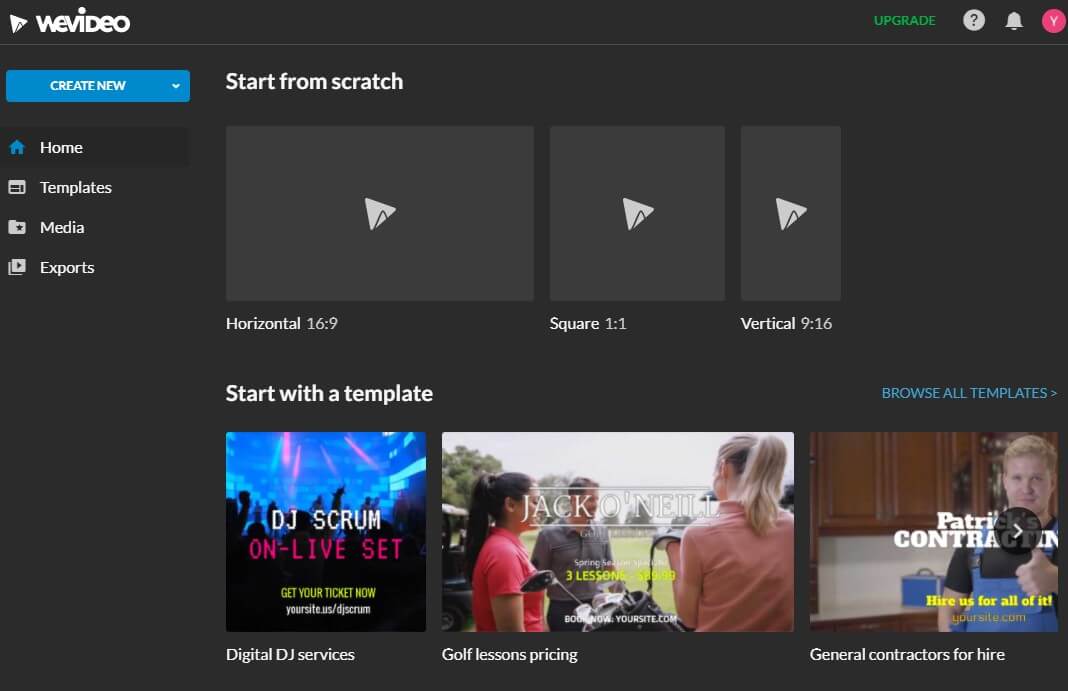This website screenshot is from WeVideo and features several navigational options and promotional templates. At the top, a tab labeled "Create New" is prominently displayed. Below this tab, there are options labeled "Home," "Templates," "Media," and "Exports." Adjacent to these, a button labeled "Start from Scratch" appears, alongside three template format options: Horizontal, Square, and Vertical. Below this section, another prompt suggests users to "Start with a Template," showcasing various sample templates such as "Digital DJ Services," "Golf Lessons Pricing," and "General Contractors for Hire."

The "Digital DJ Services" template prominently features text promoting DJ Scrum’s live set, urging viewers to get their tickets at yoursite.us/DJScrum. The background of this template depicts a vibrant nightclub scene with people dancing in dim lighting. 

The "Golf Lessons Pricing" template includes an image of golf instructor Jack O'Neill, accompanied by two or three others, seemingly engaged in a lesson. 

The "General Contractors for Hire" template shows an image of Patrick's Contracting, where Patrick is giving a thumbs up with a tagline that says "Hire Us for All of It."

On the right-hand corner of the screen, there is a prominently blacked-out "Upgrade" button with green text, flanked by a question mark icon, a bell icon, and a letter "Y" inside a pink bubble. The entire interface stands out against a plain dark gray background, providing a clear and organized layout.